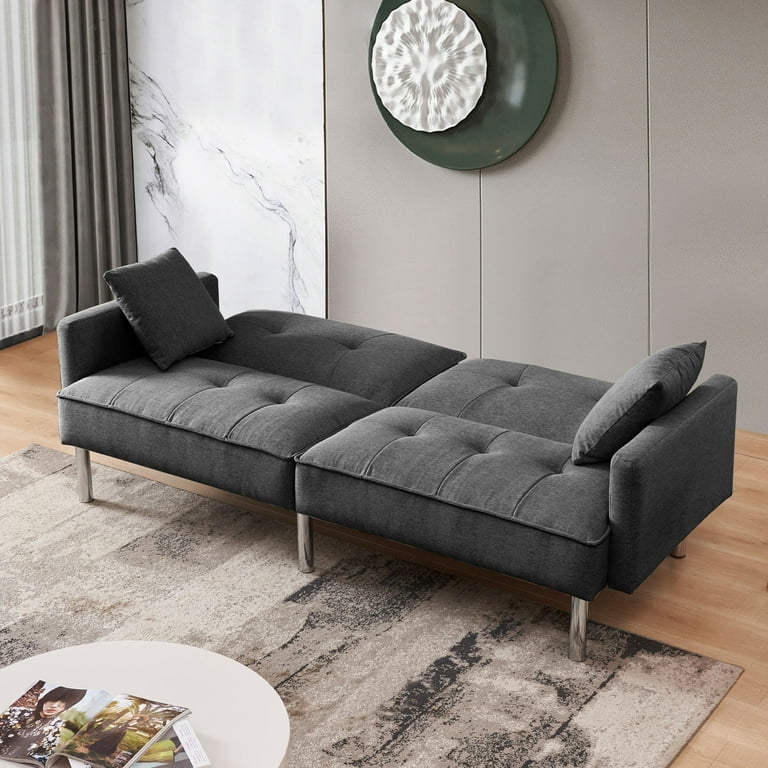The image depicts a modern living room, characterized by a neutral color scheme and bright natural light. Taking center stage is a distinctive gray couch that resembles a psychologist's lounge chair or daybed, with its back laid flat and accompanied by two pillows on either end. The couch rests on metal cylindrical legs, adding a contemporary touch. In front of the couch, there's a circular coffee table adorned with magazines. 

The floor is covered with light brown wooden planks and a tan and black rug with prominent black markings. The room features a mix of wall textures, including a marble-like white wall on the left and a gray wall on the back, which together create a sophisticated backdrop. 

Adding to the decor is an intriguing piece of artwork on the back wall, consisting of a half-sphere with a white plate attached, giving it a shell-like texture and a greenish circular motif. To the left of the image, billowing drapes frame a window, further emphasizing the room's airy and welcoming atmosphere.